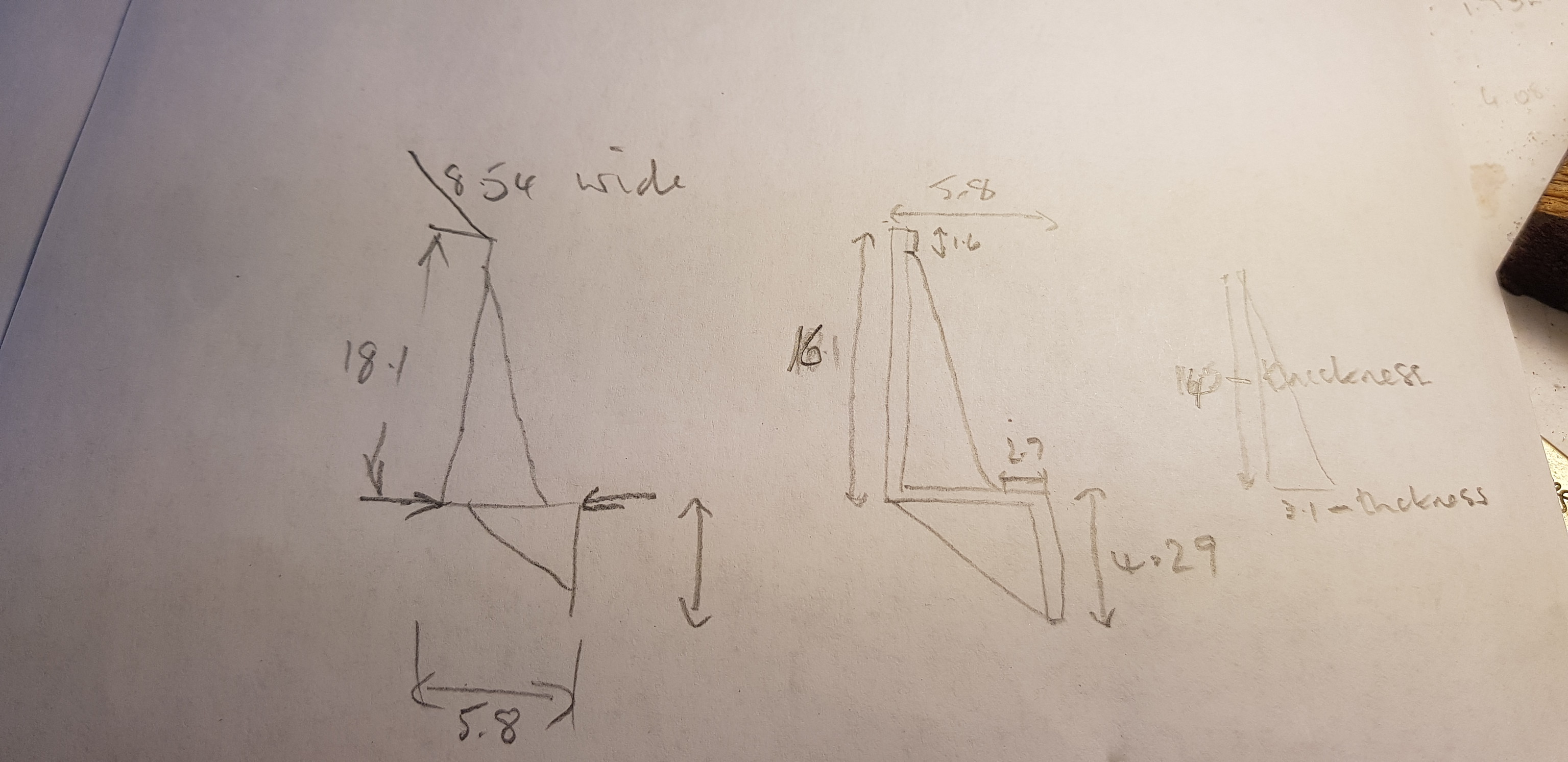The image depicts a detailed pencil sketch of architectural plans on a white sheet of paper, presumably from a sketch pad, as the edges suggest it's bound with other sheets. The main focus is a large triangle with meticulous measurements, including the top side marked as 8-1, with double-headed arrows indicating dimensions. Below the primary triangle, there's a smaller triangle, also meticulously measured with arrows pointing inward and outward. 

Adjacent to the prominent triangle, a vertical line with directional arrows displays further measurements, including a section labeled 5.8 on a graph-like diagram situated between two lines with arrows. Additional sketches include two elongated, slender triangles with measurements marked at 16-1, and underneath these, another shorter triangle annotated with 4-29. 

On the right side of the sheet lies a solitary triangle, also detailed with measurements, and several annotations repeated the term "thickness" in different sections. The sheet rests on a surface where a fragment of the floor and a piece of wood are visible on the right side, adding context to the setting in which the sketch was created.